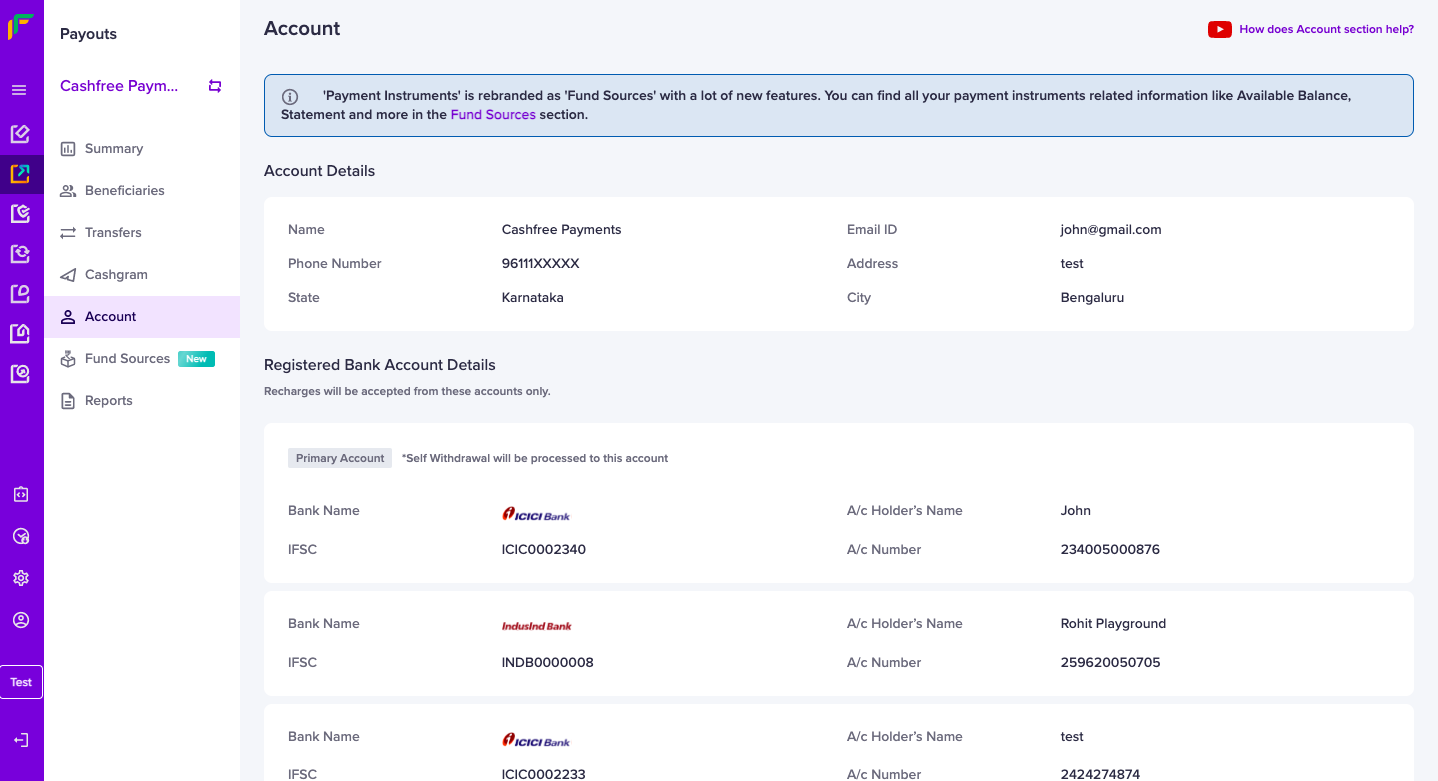This image is a screenshot of a webpage interface for managing payouts, specifically within the CashFree Payments platform. In the top left corner, the word “Payouts” is shown, accompanied by the “CashFree” logo and a truncated “Pay with M…” button.

On the left sidebar, there is a navigation menu with several options: “Summary,” “Beneficiaries,” “Transfers,” “Cashgram,” “Account” (which is currently highlighted), “Fund Sources” (with a "New" tag), and “Reports.”

To the right of this sidebar, the main header reads "Account." Directly beneath, a boxed section states: “Payment instruments are rebranded as Fund Sources with many new features. You can find all your payment instruments related information like available balance, statement, and more in the Fund Sources section."

Below this note, under the "Account Details" section, several form fields specify user data: Name, Phone Number, State, Email ID, Address, and City. Each of these fields is populated with the respective information, with “CashFree Payments” listed as the name.

Further down, a section titled “Registered Bank Account Details” notes that recharges will be accepted only from these accounts. A tab for the “Primary Account” indicates that self-withdrawals will be processed to this account. This section contains fields for “Bank Name,” “IFSC,” “A/C Holder's Name,” and “A/C Number.” Three different accounts are listed in this section, each filled with distinct information respective to those accounts.